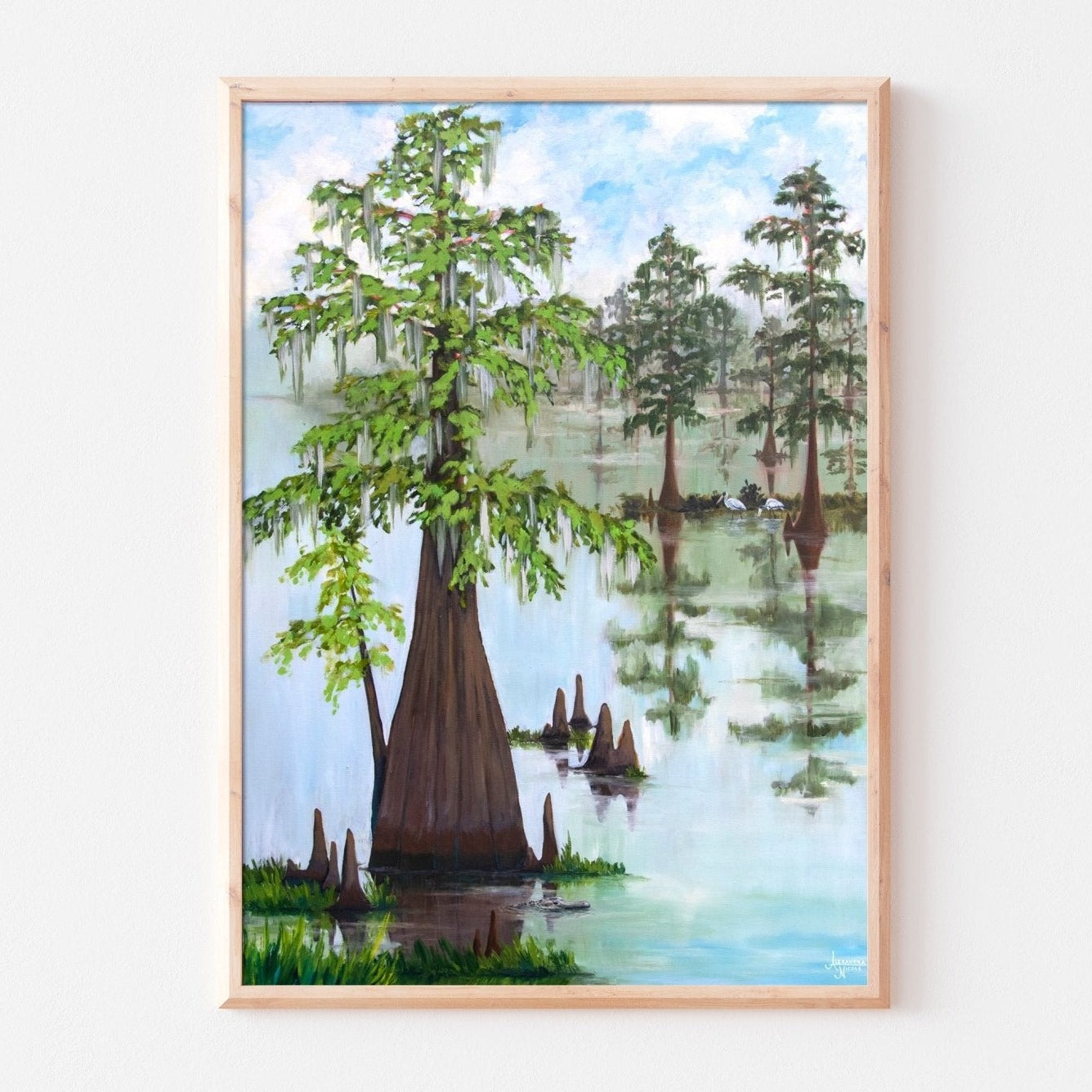A beautifully framed painting, encased in a peach-colored frame against a gray wall, captures a serene lakeside scene dominated by verdant trees. In the foreground, a prominent tree with bright green leaves stands next to patches of grass and enigmatic brown cone-shaped formations emerging from the shimmering, light blue lake. Scattered lily pads float on the serene water, where white ducks swim gracefully. The water, reflecting the scene above, mirrors the lush foliage of the trees and the bright blue and white sky dotted with clouds. The painting also features distant trees with darker green leaves and possible seagulls perched nearby. A white, unreadable signature graces the bottom of this tranquil and detailed artwork.